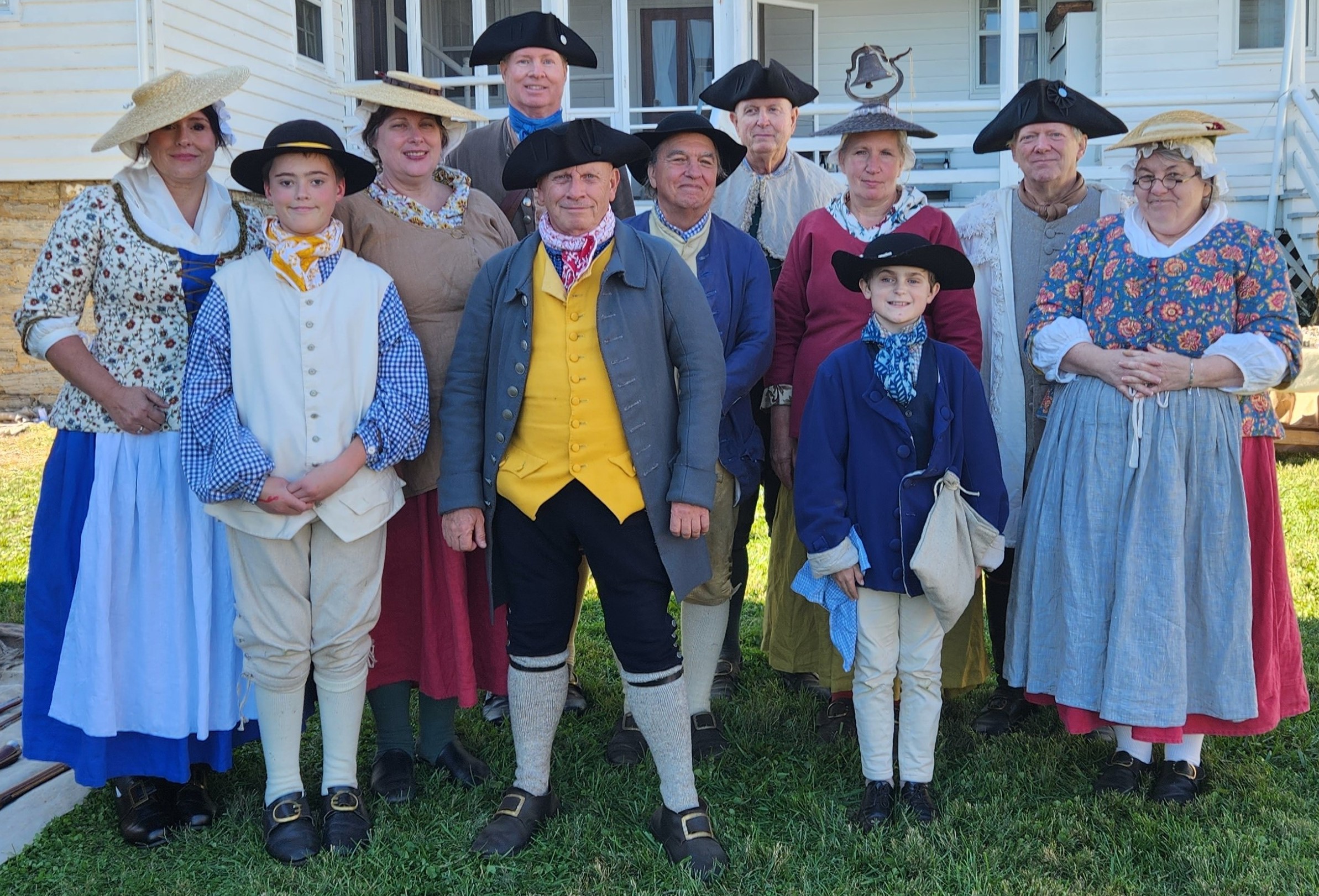This image features a group of eleven individuals—comprising four women, four men, and two young boys and a young girl—dressed in a variety of historical, pilgrim-inspired costumes. The women wear traditional, long pilgrim-type dresses accompanied by wide-brim straw hats, evoking an old-time kitchen baking scene. The men sport a mix of pilgrim and pirate-like attire, including black caps reminiscent of French army hats. Each person is uniquely dressed with varied colors, making the scene vibrant despite the historic flavor. The youngest boy, aged around 7 or 8, stands near the front clad in a blue jacket, black hat, and tan pants, holding a bag. The older boy, approximately 10 to 12 years old, is also prominently visible. They are all posed on the grassy front yard, with an old-time bell and partially visible large white house with windows forming the backdrop, evoking a sense of a heritage day celebration. The entire group appears to be enjoying themselves, adding to the lively and festive atmosphere of the scene.